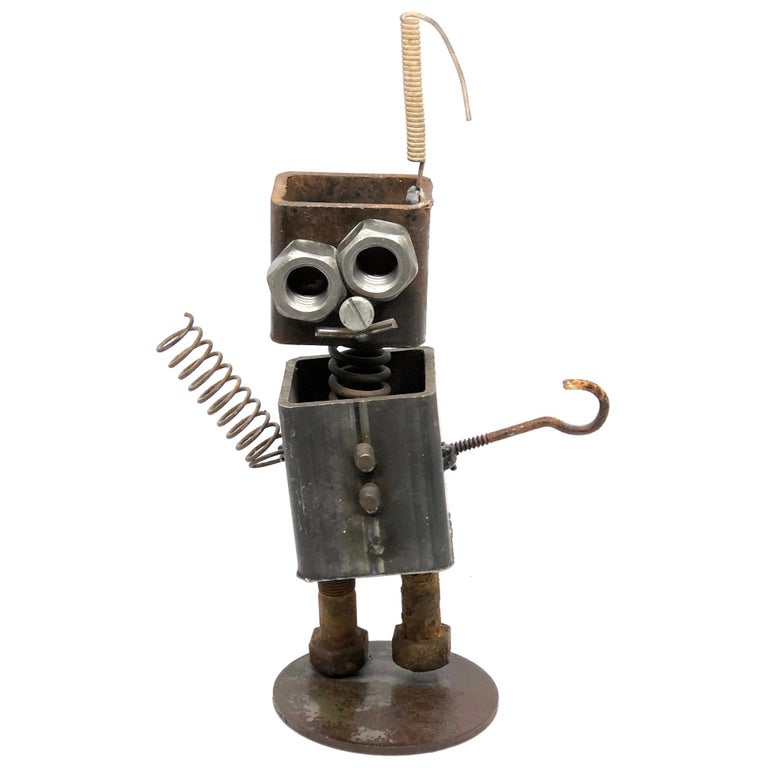This detailed image depicts a meticulously crafted sculpture of a makeshift robot, assembled from various scrap metals. The robot stands on a circular metal disc, with feet fashioned from hexagonal bolts. Its body is a cut rectangular steel beam adorned with two prominent screws acting as buttons on the front. The left arm is a flexible spring, while the right arm is a sturdy screw hook. The neck is an extended coil rising from the body to support the head. The head itself is a square cutout resembling a pipe, featuring eyes formed from nuts, a screw for the nose, and a curved wire forming the mouth. Atop the head, a tightly wound spring extends, possibly representing an antenna or hair. The robot's overall appearance combines dark metal tones with shiny silver highlights on the eyes and nose, all set against a plain, white background.